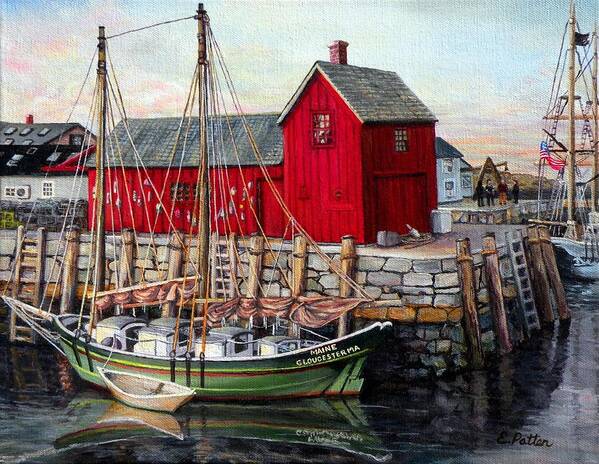This painting, potentially an oil painting by E. Patton as indicated by the watermark in the bottom right, depicts a serene waterfront scene at a pier. Dominating the foreground is a green boat labeled "Maine Gloucester MA," moored at the stone dock. Adjacent to the boat, a small emergency vessel floats beside it. The dock features a ladder leading down to the boat, emphasizing the connection between the land and the watercraft. 

In the mid-ground of the artwork stands a prominent red barn-like structure with a grayish roof and a brick smokestack. This two-level building appears to serve as a storage or supply facility, possibly for emergency rations for nearby ships. Directly behind this red barn is a smaller White House, surrounded by four individuals who seem engaged in conversation. An American flag flutters beside another boat, enhancing the scene's sense of place.

Further adding to the depth of the painting, a distant tower can be seen on the horizon under a blue sky tinged with hints of orange. The overall atmosphere is peaceful and clear, capturing a moment of daily life at a bustling waterfront in Gloucester, Massachusetts.